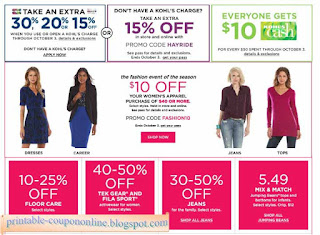This image features a promotional page brimming with various coupons and discounts. At the top, a bold heading announces, "Take an Extra 30%, 20%, or 15% Off." Below it, another section states, "Don't Have a Kools Charge? Take an Extra 15% Off," accompanied by the promo code "HEY RIDE." Adjacent to this is a green-bordered box with the offer "Everyone Gets $10 Kools Cash." The "Kools Cash" text is prominently displayed in white over a green background that mimics the design of a dollar bill.

Further down, a strikingly pink text highlights "The Fashion Event of the Season - $10 Off," alongside another promo code. Surrounding these texts are images of women showcasing fashion items like jeans and pink tops, drawing attention to the clothing offers.

Beneath these visuals, additional coupons provide further savings: "10-25% Off Floor Care," "40-50% Off TEK, Glare, and Phyla Sport," "30-50% Off Jeans," and a mix-and-match deal priced at $5.49. The page concludes with a logo at the bottom, suggesting that the source of these deals is "printablecoupons.blogspot.com," potentially a coupon aggregation website. The overall design features a clean white background accented by various colored texts, including blue and purple, creating a visually engaging and organized layout.